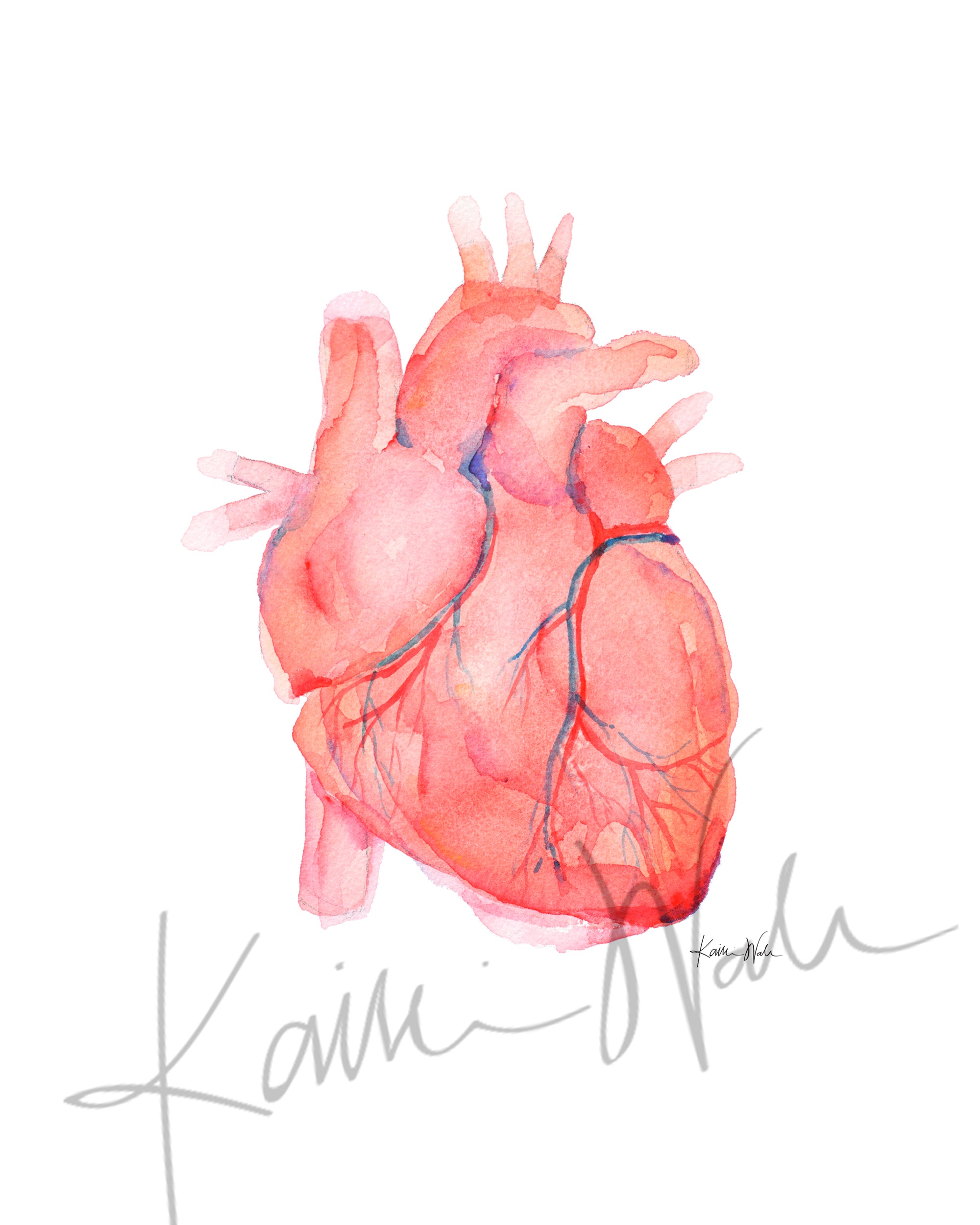This artwork is a detailed watercolor and ink illustration of the human heart, signed in cursive by an artist whose name appears to be K-A-I-R-E N-A-D-I. Set against a white background, the piece employs an array of colors—white, red, blue, pink, purple, and various shades of these hues—to depict the heart and its intricate network of veins and arteries. The colorful threads of red and blue weaving through the ventricles lend the work a semi-realistic yet artistic flare. While not hyper-realistic, the artist has meticulously crafted the details, paying careful attention to the heart's anatomical features. The piece is realistic enough to evoke the appearance of an actual heart, but its artistic elements make it clear that this is a drawn and painted representation, not a photograph.